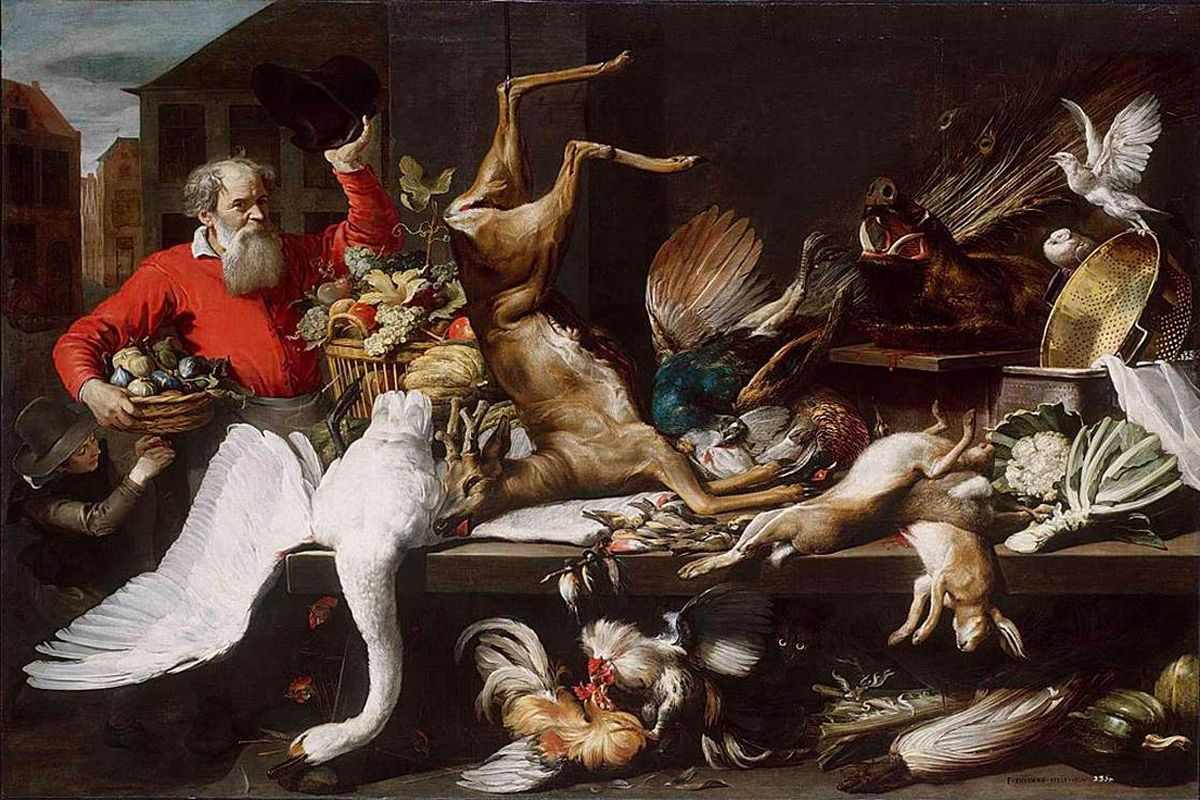The illustration, reminiscent of 19th or early 20th-century artwork, is a highly realistic depiction of a market scene laden with the aftermath of a hunt. On the left side, a bearded, balding man in a red shirt with a white collar is depicted raising a black hat in his left hand, as if in greeting. His right arm cradles a basket filled with circular vegetables. At his waist, a small child dressed in a black hat and vest reaches up towards him. The background to the left consists of silhouetted buildings against a pale blue cloudy sky, while the top right of the image is dominated by a dark, blank wall.

In the foreground, a long wooden table stretches almost entirely across the scene, heaped with an assortment of dead animals. A deer rests with its chest and neck on the table, its rear hoisted by a string into the sky. Nearby, a sprawling white swan's body lies on the table, its head and one wing drooping onto the floor, its black legs sticking up. Beside it, a boar occupies a raised section of the table, bleeding, surrounded by two hares and numerous birds. Additional dead animals populate the table, including foxes that appear to teeter off the edge. Amid the deceased fauna, live chickens—one gold and one black and white—flit around the table's base.

Scattered around the main table are wicker baskets brimming with fruits and various smaller vegetables, enhancing the scene's market atmosphere. The intricate detailing and the interplay of life and death on the table captures a vivid moment frozen in time, blending the bustling energy of a marketplace with the somber reality of a hunter's haul.